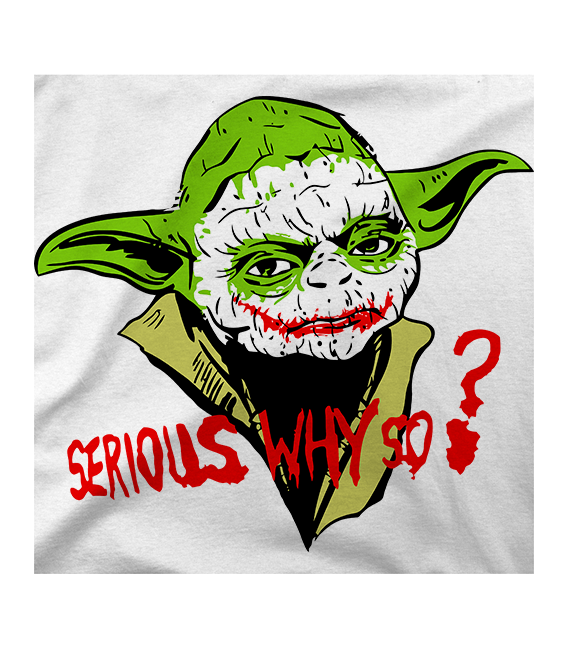The T-shirt features a striking image that blends elements of Yoda from Star Wars with the iconic appearance of the Joker from DC Comics. The figure has Yoda’s distinctive green skin and long ears, yet sports white face makeup with many black lines, and red lips that extend into a menacing Joker-like smile. His eyes are a vivid green. Yoda's hair is also green, and he wears a mustard green outfit with a long collar. This detailed mash-up image is printed on a white T-shirt. Below the image, in bold red text, is the phrase "Serious? Why so?" with a question mark, playing on the Joker’s famous line and further emphasizing the fusion of these two characters.